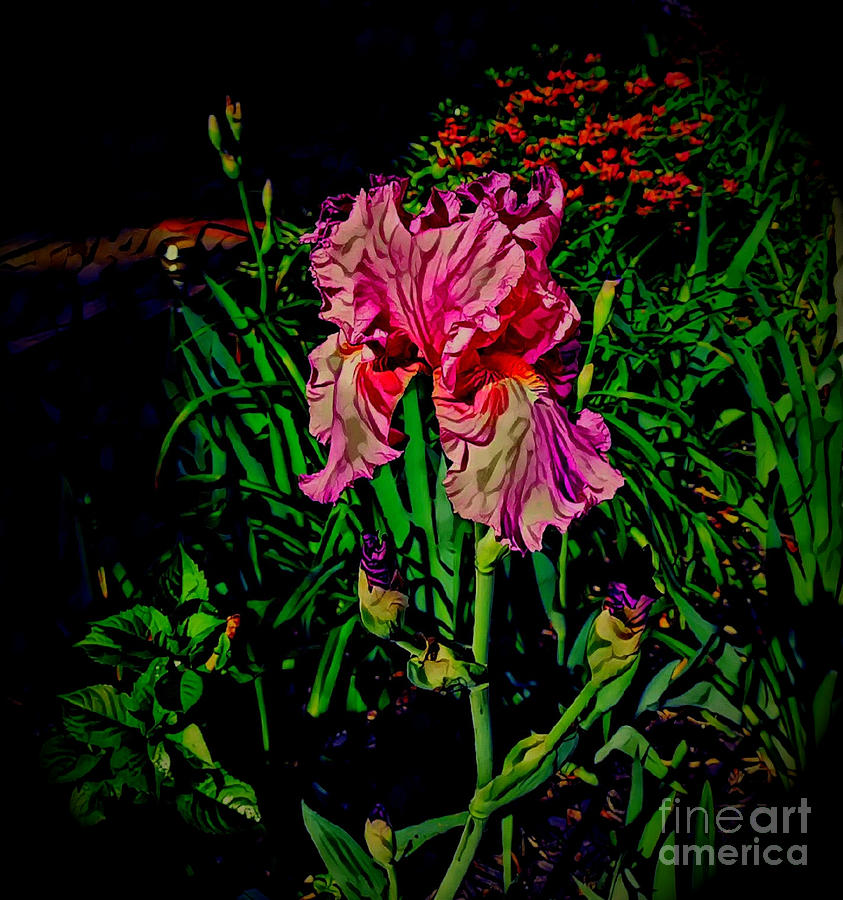This highly detailed artwork, likely a drawing or painting, features a vibrant, blooming flower as its central focus. The artwork's lower right corner is marked with the text "Fine Art America" in white letters of varying sizes and fonts. The centerpiece flower, an exquisite mix of pink, red, white, and purple hues, boasts sprawling petals that extend upwards and droop slightly, resting on a sturdy green stem amidst surrounding green foliage that adds depth and texture. The composition is enriched with complementary floral elements, including budding small purple flowers and petite red blooms interspersed throughout. Surrounding the main flower on the left, a variety of green grasses and stems intertwine with orange flowers, creating a lush and colorful scene. The dark background, suggestive of a nighttime setting, contrasts sharply with the vivid flora, enhancing the overall vibrancy of the piece and contributing to its dynamic visual appeal.